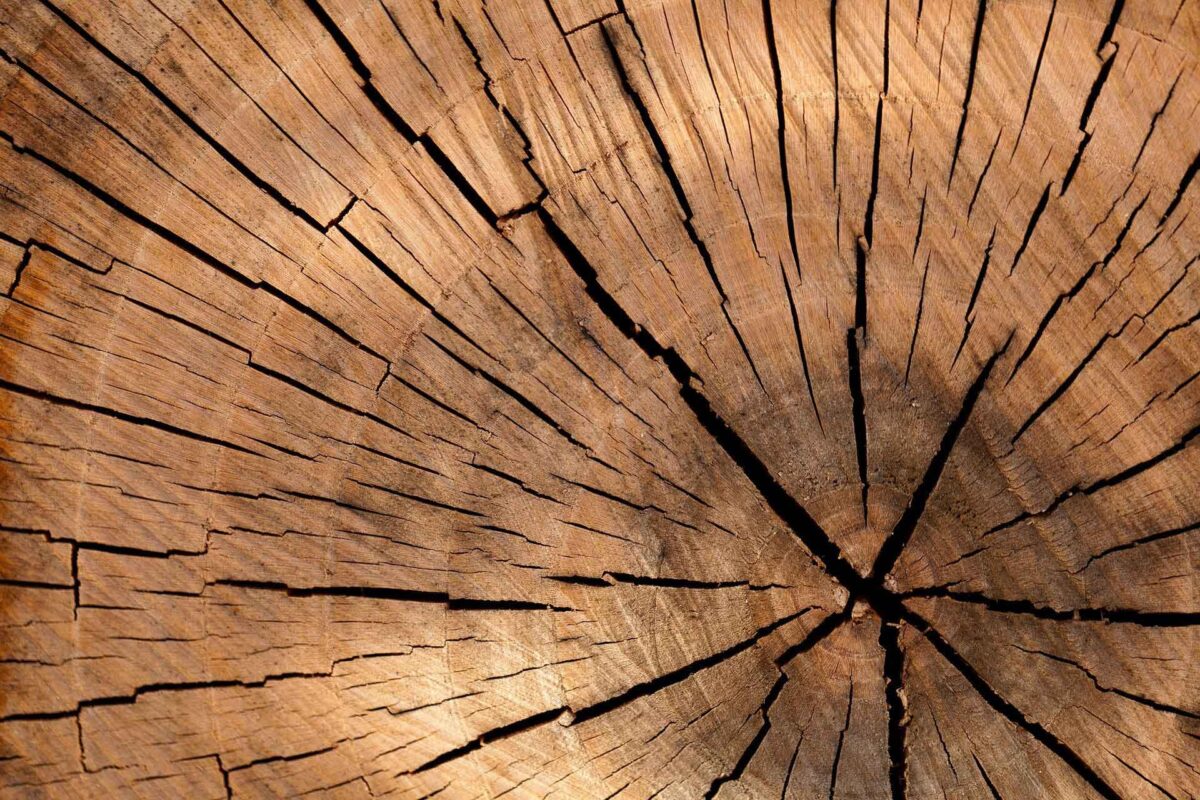The image depicts an extreme close-up of the cross-section of a cut-down tree trunk, occupying the entire frame. The stump, appearing old and dry, is a study in shades of brown and tan, with notable color variation; light browns dominate parts of the wood, while there are darker, nearly black hues concentrated in the deep, wide cracks that traverse the stump horizontally and radiate outwards in a starburst pattern. These cracks, born from the drying process, are particularly pronounced towards the center of the stump and become narrower towards the edges. The tree rings, numbering between 13 to 15, are clearly visible amidst the splinters and cracks, highlighting the tree's age. The center of the cross-section is slightly offset towards the bottom right of the image, illustrating the intricate, aged texture of the wood.